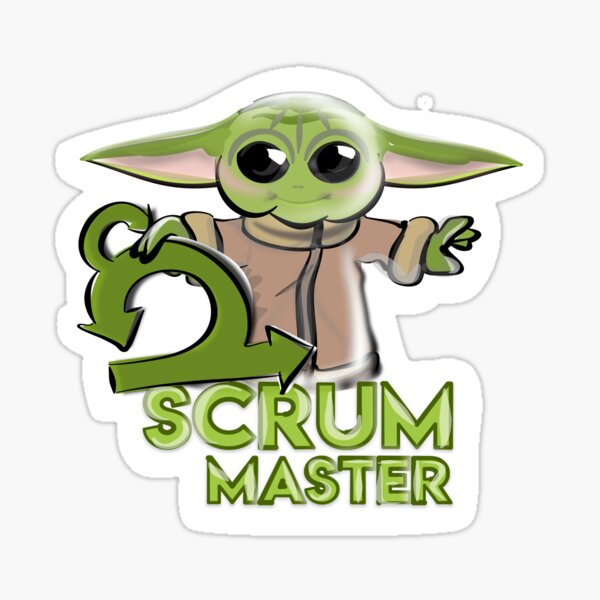The image features a detailed drawing of Yoda from Star Wars, dressed in a brown robe with thick arm cuffs against a white background. Yoda, characterized by his wide dark eyes and horizontally protruding large green ears, stands with his arms extended to each side and holds a circular symbol composed of three arrows pointing in different directions. His face is marked with a series of vertical and horizontal lines, and he has grayish wide eyebrows. Below Yoda, the green text "Scrum Master" stands out, highlighted by a darker green outline. The entire drawing is bordered by a gray line, giving it the appearance of a sticker or bumper sticker.